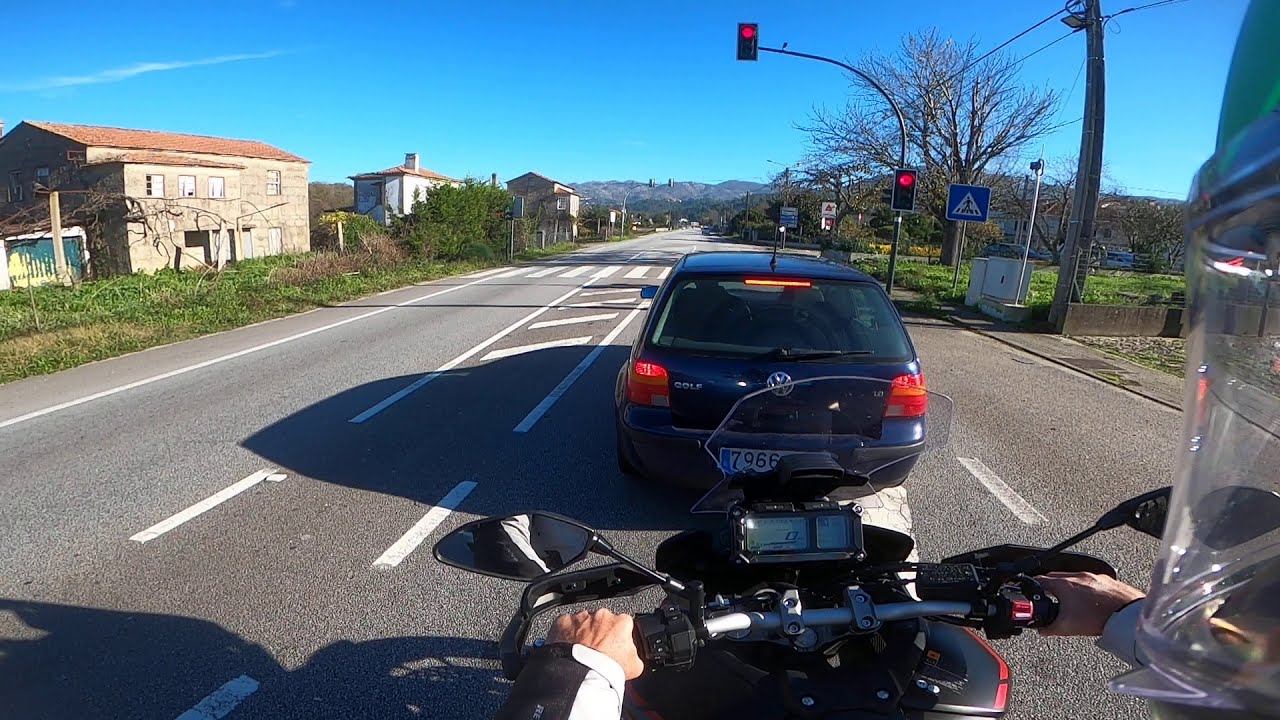This photograph, taken from the perspective of an individual riding a motorcycle, offers a detailed view of both the rider's and their surroundings. The rider's white-gloved hands grip the handlebars, while a portion of their helmet and the attached clear face shield are visible on the right side of the image, suggesting that a GoPro is mounted there. The speedometer of the motorcycle reads zero, indicating that the rider is stopped at a red light. Directly ahead, a blue Volkswagen Golf, identifiable by its European license plate displaying the partial number 7966, is also halted.

The scene is set on a two-lane road with white-striped crosswalks and a central bike lane, hinting at a European setting. The left side of the road features rundown houses, possibly reminiscent of European or Italian architecture, surrounded by bushes and a fence. To the right, the roadside is dotted with various blue road signs, trees with sparse foliage, and utility infrastructure, including an electrical line and transformer box. The blacktop road, accompanied by an array of details, paints a vivid picture of a typical, perhaps slightly rustic European street.